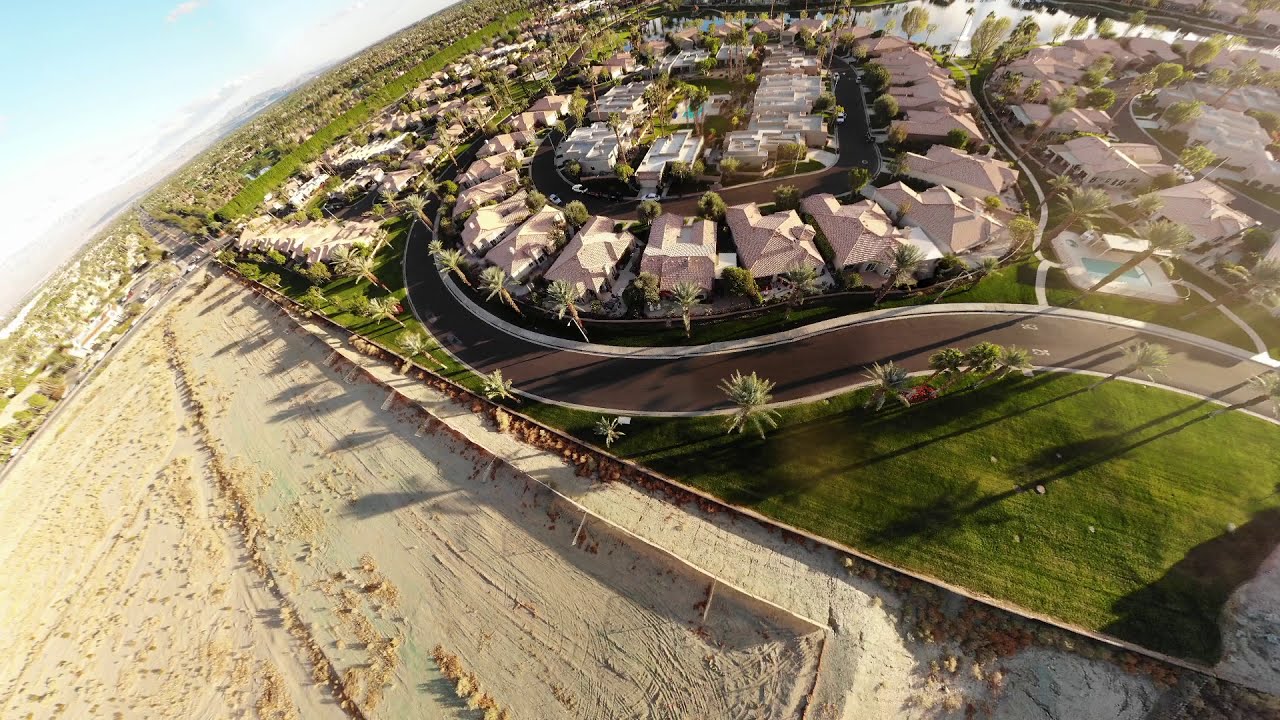This overhead drone photo captures a tightly packed housing development in what appears to be a desert or sandy area. The image, slightly tilted, shows a freshly paved semicircular road winding through closely wedged houses. Sand is noticeable in the lower left corner, contrasting with the green grass patches and palm trees scattered around the neighborhood. Some houses have swimming pools, and a white fence is visible in the upper right corner, marking the boundary of the development. The overall setting is sunny, emphasizing the arid, desert-like surroundings of the neatly structured and modern-looking houses.